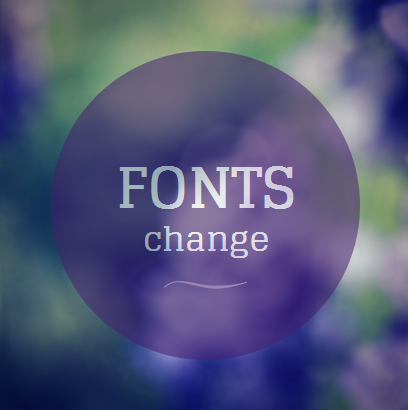The image is a full-color, square photograph with a completely out-of-focus background that features a variety of colors including greens, whites, blacks, blues, and purples. At the center of the image, there is a dominant light purple circle that occupies roughly half of the entire space. Inside this circle, two white words are prominently displayed: "FONTS" in larger, all-capital letters at the top, and "change" in smaller, lowercase letters at the bottom. Below the two words, a decorative white swoopy or wavy line adds an additional visual element. The varied background colors include green, blue, and purple, enhancing the light purple circle's prominence in the image.